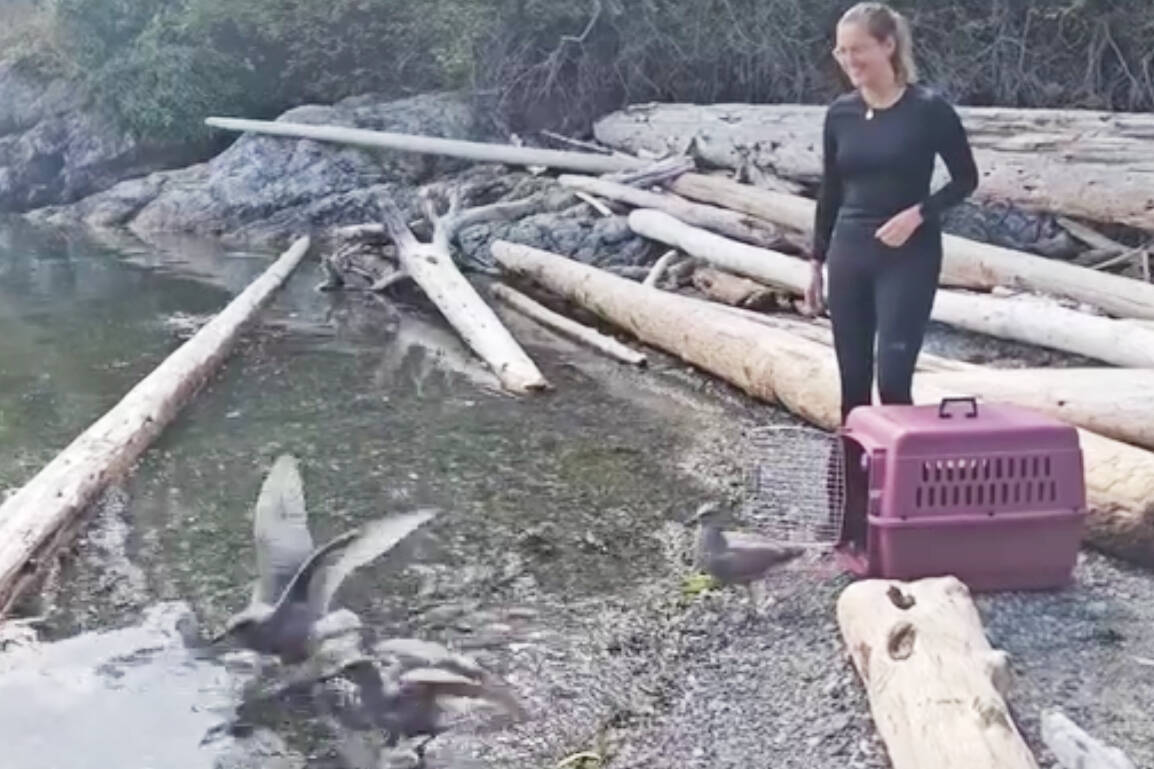The image depicts a smiling blonde woman wearing glasses and a black wetsuit-like outfit, consisting of black spandex pants and a long-sleeve shirt. She is standing beside a pink portable pet cage with an open door, from which three white birds, likely ducks, are emerging. One bird is already in flight, while two others are walking out of the cage. The scene is set outdoors in a bright, forested area. The woman is standing on a gravel shore next to a shallow stream, surrounded by long, fallen tree logs and green-brown brush. The left-hand side of the image shows the green water of the stream, which recedes towards her feet. The background is filled with more trees, emphasizing the natural and serene environment where the birds are being released back into the wild.